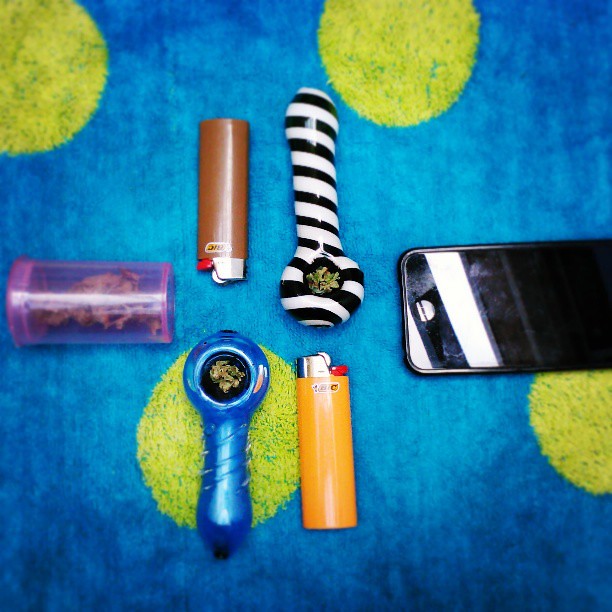The photograph captures a square-shaped scene set on a blue background, possibly a rug, blanket, or beach towel with a fuzzy texture. The blue fabric shows variations in color, being lighter at the center and darker at the edges, possibly due to lighting, and features green-yellow circles. Arranged in a layout resembling a plus sign, the objects displayed include a black smartphone positioned at the right, extending from the three o’clock position towards the center. To the left, around the nine o'clock position, there's a transparent pink container filled with marijuana. In the vertical axis, an orange Bic lighter with black "BIC" text, a red button, and a silver metallic lighting mechanism sits below a blue marijuana pipe with weed in the bowl. Above, at the top center, there's an upside-down brown Bic lighter near a white and black striped marijuana pipe that is also upside down with weed in the bowl. The overall arrangement and objects suggest a casual or youthful setting, possibly intended to be shared on social media.